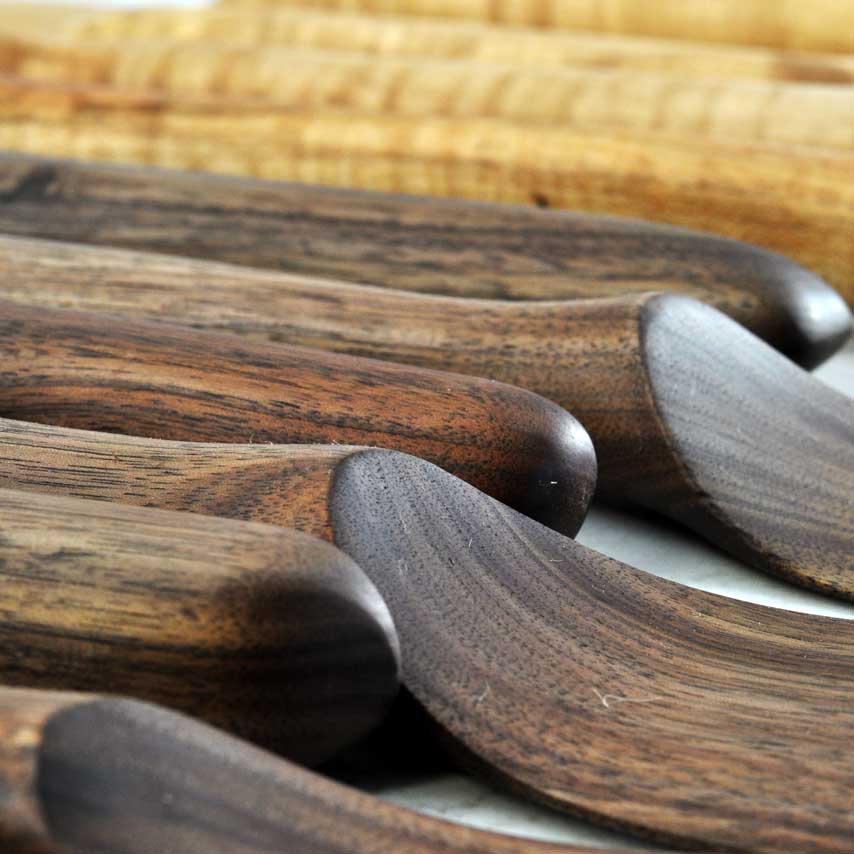The image shows a close-up of six intricately worked wooden implements laying next to each other on a gray table or mat. The meticulously carved pieces vary from curved, spatula-like ends to rounded handle ends, suggesting they are part of a set of wooden tools or utensils. The wood features a dark, swirly, and smudged grain pattern, indicative of a staining process, possibly accompanied by slight burning, adding to the rich, dark character. The wood has been sanded to a smooth finish, contrasting with some untreated lighter wood visible in the background. The arrangement moves horizontally from left to right, with the closest wood pieces appearing sharp and detailed, showing off their finely worked grain, while the wood in the background becomes progressively blurred and lighter.